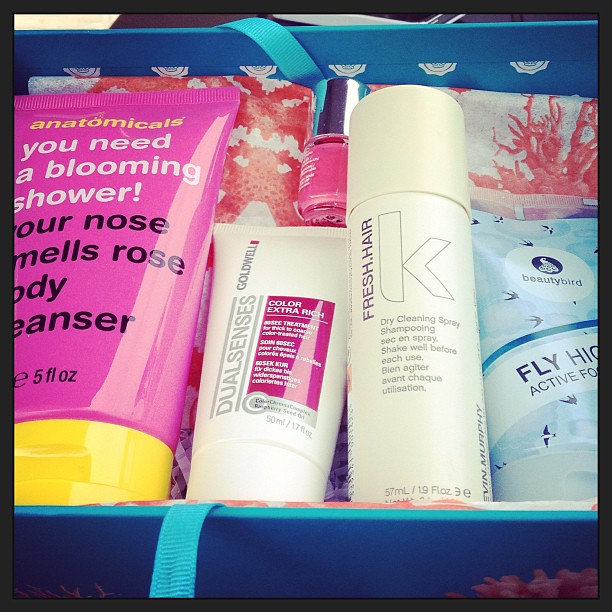This photograph features an unboxing of a meticulously arranged care package, likely intended for a female recipient, housed in a blue cloth basket accented with pink at the bottom right-hand side. The basket is adorned with a ribbon and white logos inside, giving it an Instagram-worthy aesthetic.

Inside, there are five key beauty products arranged vertically. On the left, there's a vibrant pink tube of Anatomicals "Your Nose Smells Rose" body cleanser, distinguished by its yellow screw cap. Next to it sits a smaller white tube labeled "Color Extra Rich," suggesting it is a hair treatment product. Positioned further right is a predominantly white bottle of Fresh Hair K dry shampoo, featuring purple lettering. Adjacent to this is a blue package from the Beauty Bird brand, though the specific product is unclear. Finally, nestled at the back is a petite jar of pink nail polish with a silver lid.

The varied colors—pink, white, blue—and the mix of functional cosmetic items like cleansers and nail polish create a visually appealing and thoughtful beauty kit.